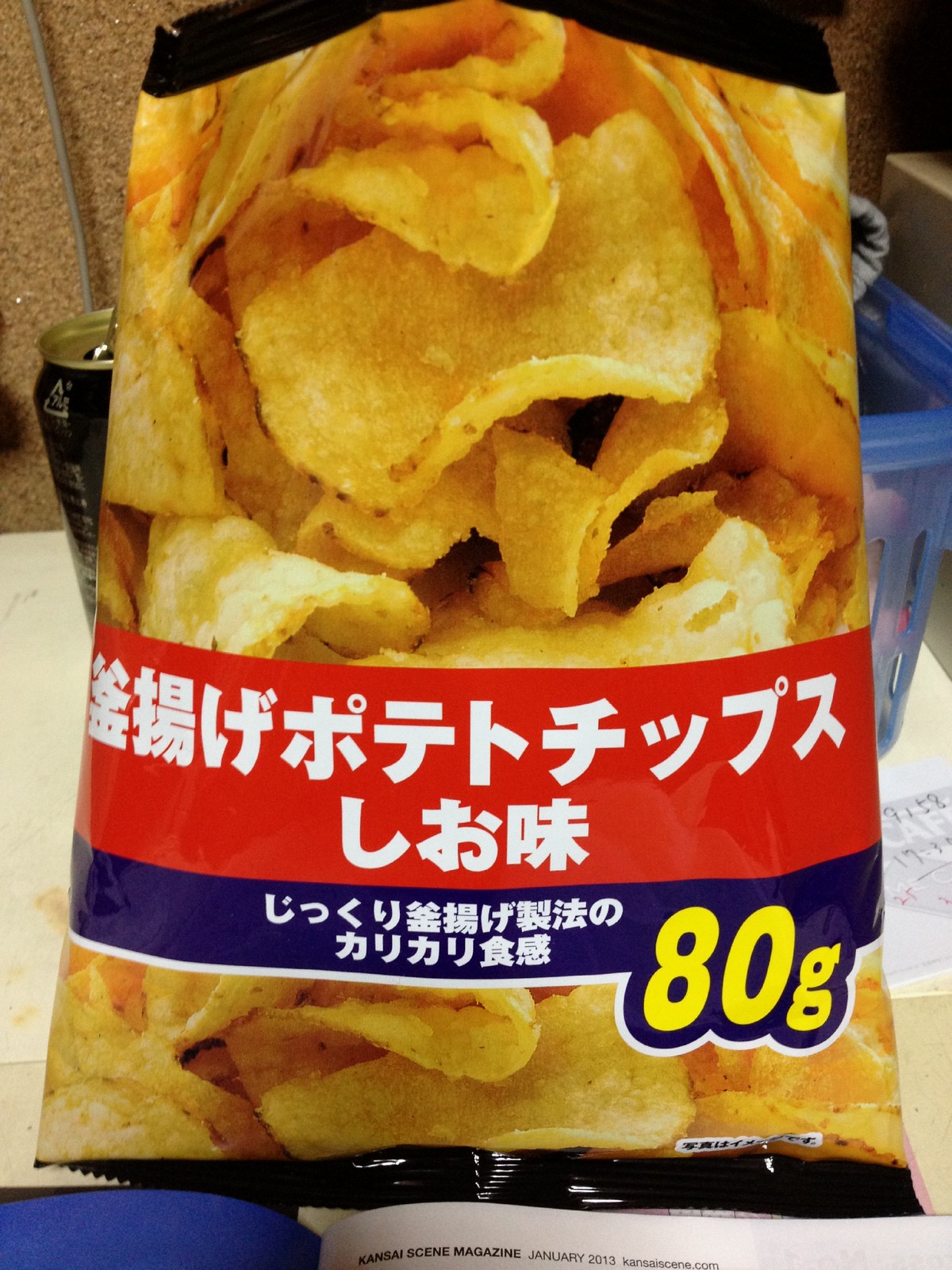The photograph depicts a bag of plain, golden-brown kettle chips prominently displayed against a background featuring various objects. The bag itself showcases a real photograph of the chips, which are round, crunchy, and folded, without any visible seasoning. The packaging features large white Japanese characters over a red border and a blue line with additional smaller kanji characters. The bottom right corner of the bag displays "80G" in bold yellow text. The bag is set on a countertop, with a black can with a golden lid, a blue basket, and a white paper with writing in the background. The setting is further framed by a cork board and a glimpse of a book's top edge, adding context to the scene.